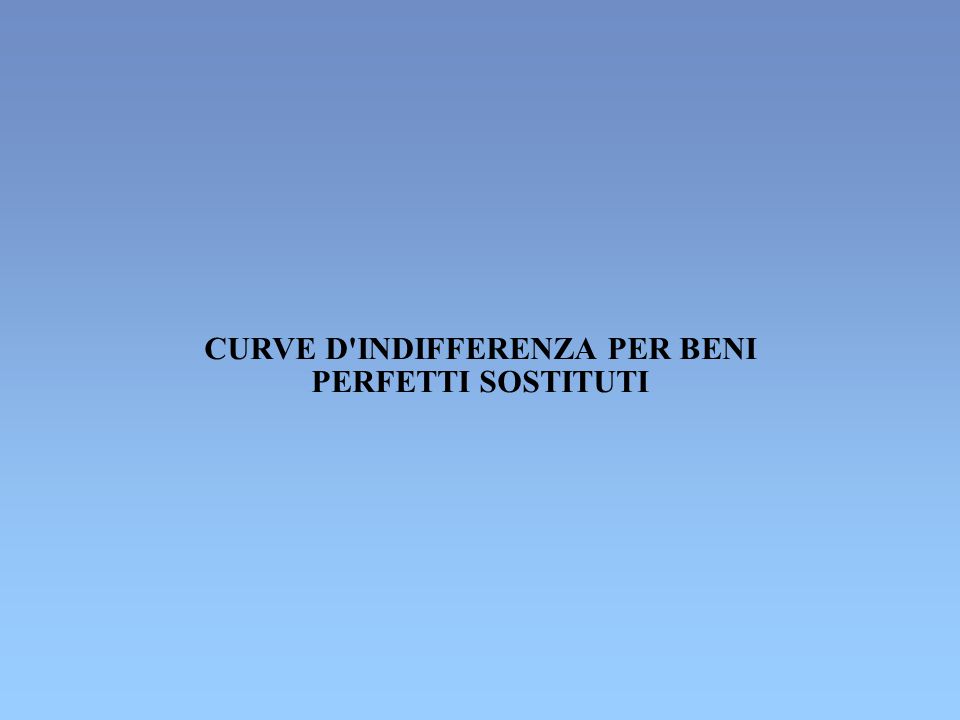The image features a simple and elegant design with a blue gradient background rectangle transitioning from an ocean blue at the top to a lighter blue at the bottom. Positioned centrally in the image is black text in a serif font. The text is in Italian and reads "CURVE DI INDIFFERENZA PER BENI" on the first line and "PERFETTI SOSTITUTI" directly below on the second line. The black uppercase letters are neatly centered both horizontally and vertically within the rectangle, creating a balanced and refined visual. There are no other images, people, or objects present in this design—it focuses solely on the gradient background and the prominently displayed text.